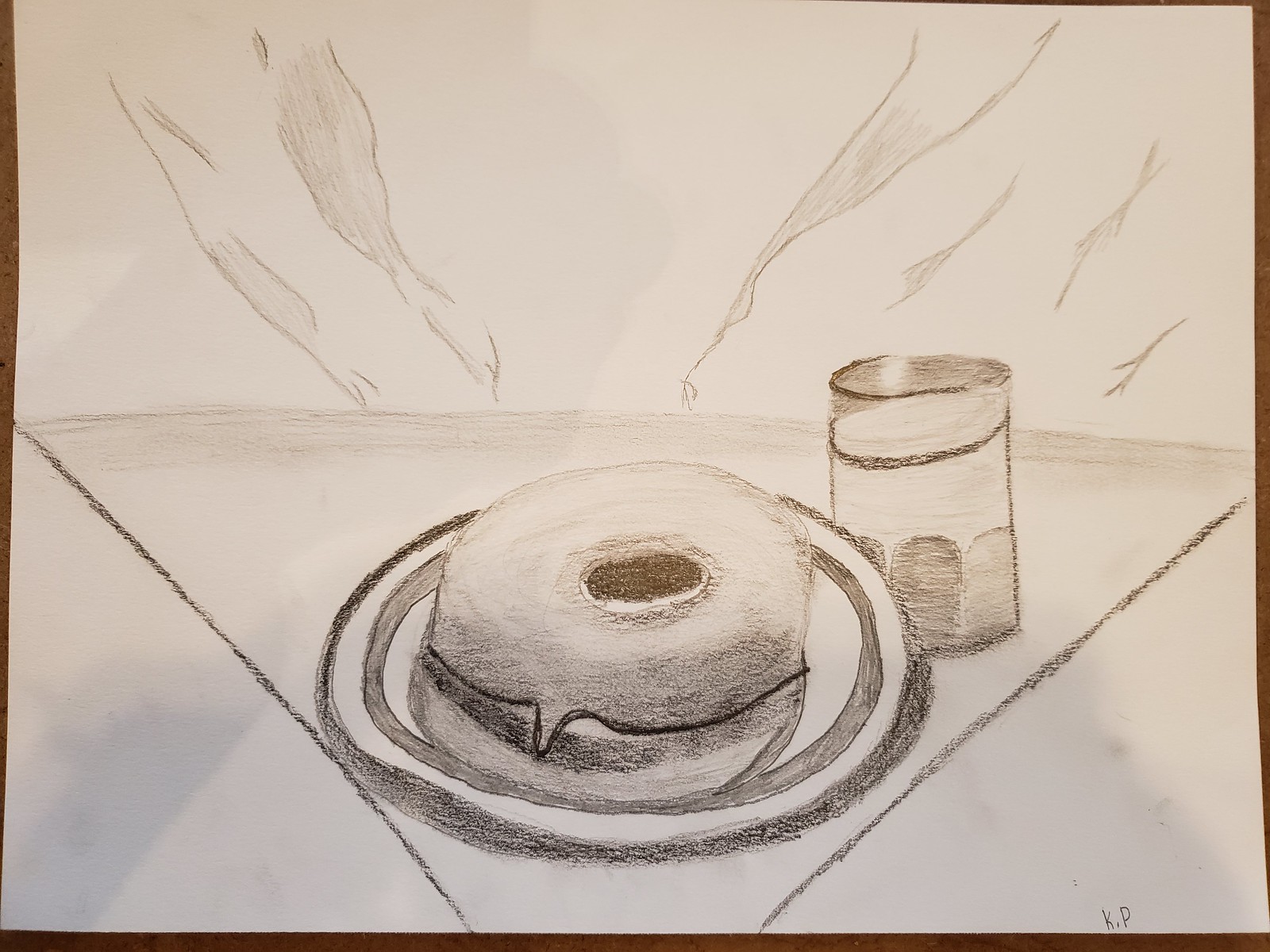This is a meticulously crafted black-and-white charcoal sketch, signed "K.P." in the bottom right-hand corner, drawn on a piece of white paper. The illustration captures a simple yet evocative scene of a breakfast table. Centered in the composition is a plate holding a bagel breakfast sandwich, characterized by its distinct hole in the middle, hinting at its bagel nature. Accompanying the sandwich is a full glass, the contents of which remain unspecified due to the monochromatic medium. The predominant shades in the image are tones of black and varying intensities of grey, effectively conveying texture and depth against the stark white background.